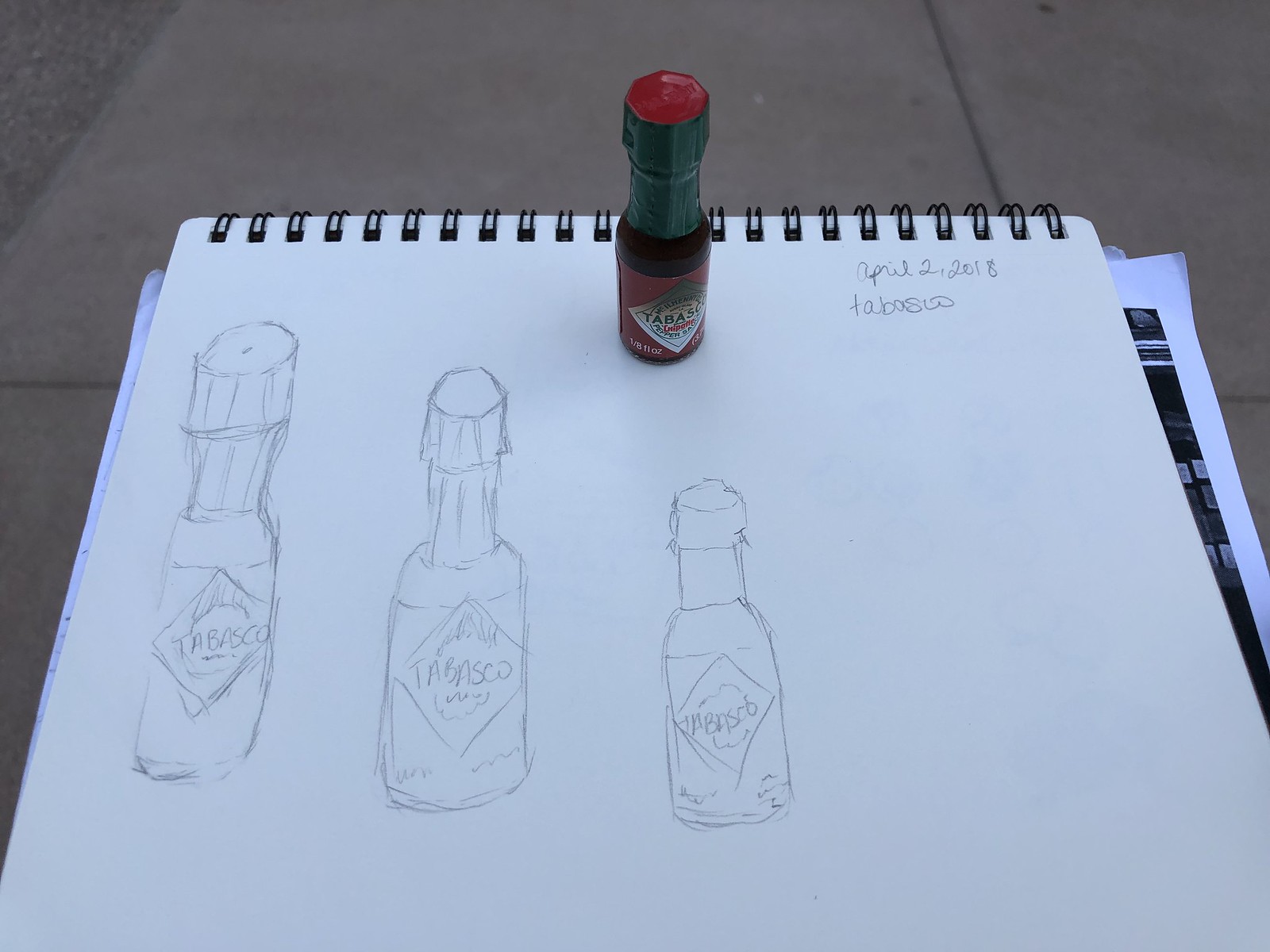This detailed caption provides a thorough description of the image:

"The sketchbook displayed in the image features three meticulously drawn sketches of a small Tabasco sauce bottle, a quintessential hot sauce known for its distinct red and green bottle with a red cap. These pencil sketches vary in size, gradually decreasing from a larger representation to a smaller one, occupying a little over a quarter of the page. The top of the spiral-bound sketchbook is visible, resting on a surface that reveals hints of a cement walkway and possibly some gravel in the top left corner. The date 'April 2nd, 2018' is clearly inscribed on the page, accompanied by the word 'Tabasco' listed beneath the sketches. Additional images or printouts seem to be tucked into other pages of the sketchbook, indicating a cluttered yet creative workspace."